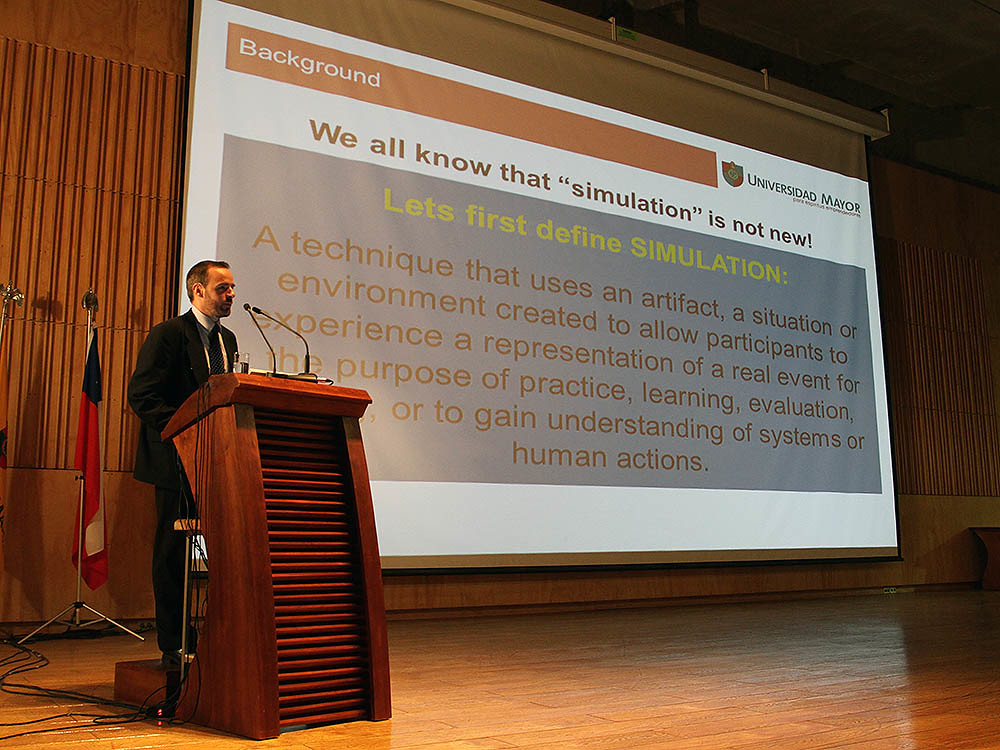In this detailed photograph from a conference or auditorium, a middle-aged Caucasian man is giving a PowerPoint presentation. He is standing behind a wooden podium equipped with two microphones and a glass of water, against a backdrop of a wooden stage and brown wooden walls. The man, who has short graying hair and a very short beard, is dressed in a black business suit with a striped tie and a white shirt. Behind him, there is a folded flag on a stand and a large canvas screen projecting his presentation. The slide, titled "Background" in a white font on a rust-colored rectangle, belongs to a presentation that prominently features text discussing the definition and application of simulation. Notably, the screen displays the logo "Universidad Mayor," suggesting the event is associated with a Spanish-speaking university. The slide reads, "We all know that simulation is not new. Let's first define simulation, a technique that uses an artifact, a situation, or environment created to allow participants to experience a representation of a real event for the purpose of practice, learning, evaluation, or to gain understanding of systems or human actions."